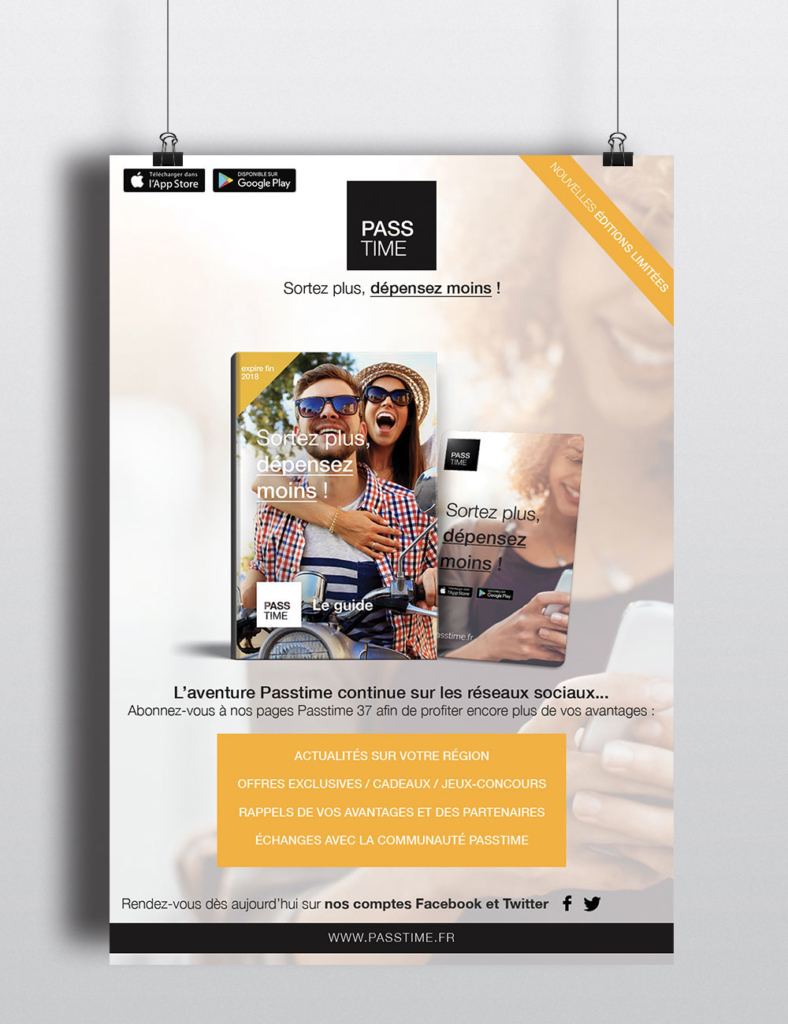The image depicts an advertisement written in French, prominently titled "Past Time." The ad appears to be a poster, hanging from two black clips connected by a black string, against a light grey background. In the top right, a diagonal orange bar states "Nouvellas Editions Limites," while a black square at the top displays "Past Time" in white font. In the upper left corner, symbols for the Apple App Store and Google Play are visible. The center of the ad features a vibrant image of a man and woman riding a motorcycle, both smiling and wearing sunglasses, with the phrases "Sortez plus, Depensez moins, Past Time" accompanying the photo. Another image below this shows a woman holding her phone, with similar text next to it. The ad includes a call-to-action indicating social media presence with the phrase, "L'Aventure Past Time continue sur les réseaux sociaux," and contains a gold square with additional French writing. The bottom part of the ad features logos for Facebook and Twitter, along with the website address "www.pastime.fr."